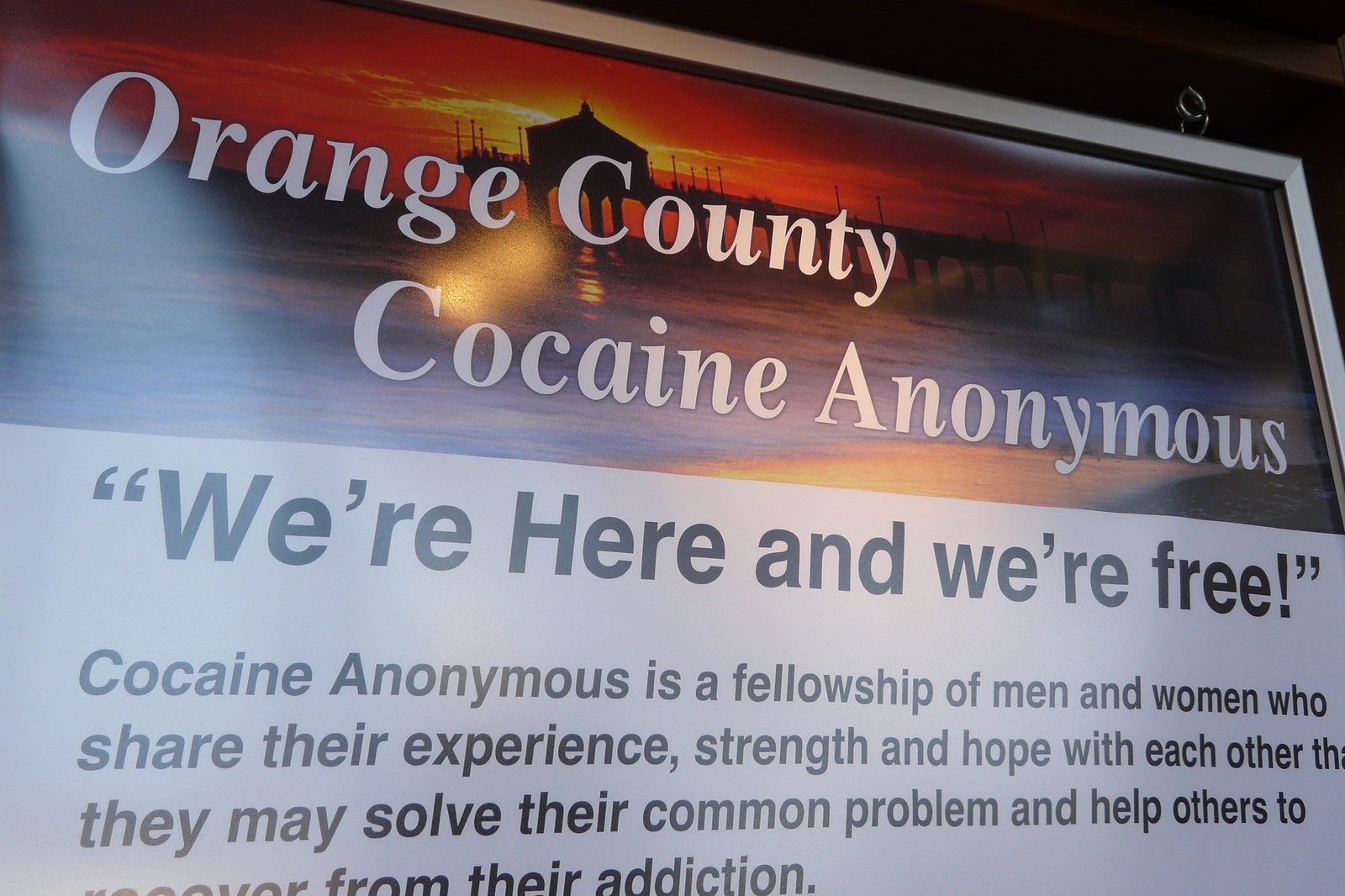The image depicts a full-color, informational billboard for Orange County Cocaine Anonymous. The sign prominently features a serene night scene with a picturesque view of a pier, complete with a building at its end and an orange and yellow sky marking either sunrise or sunset. The tranquil backdrop is accentuated with the sun partially hidden behind the building, casting a peaceful glow. In large, white letters at the top, it reads "Orange County Cocaine Anonymous." Below this, in bold white letters within parentheses, the slogan "We're here and we're free!" stands out against a white background with black text. Further down, the sign provides information about the organization, stating, "Cocaine Anonymous is a fellowship of men and women who share their experience, strength and hope with each other that they may solve their common problem and help others to recover from their addiction."